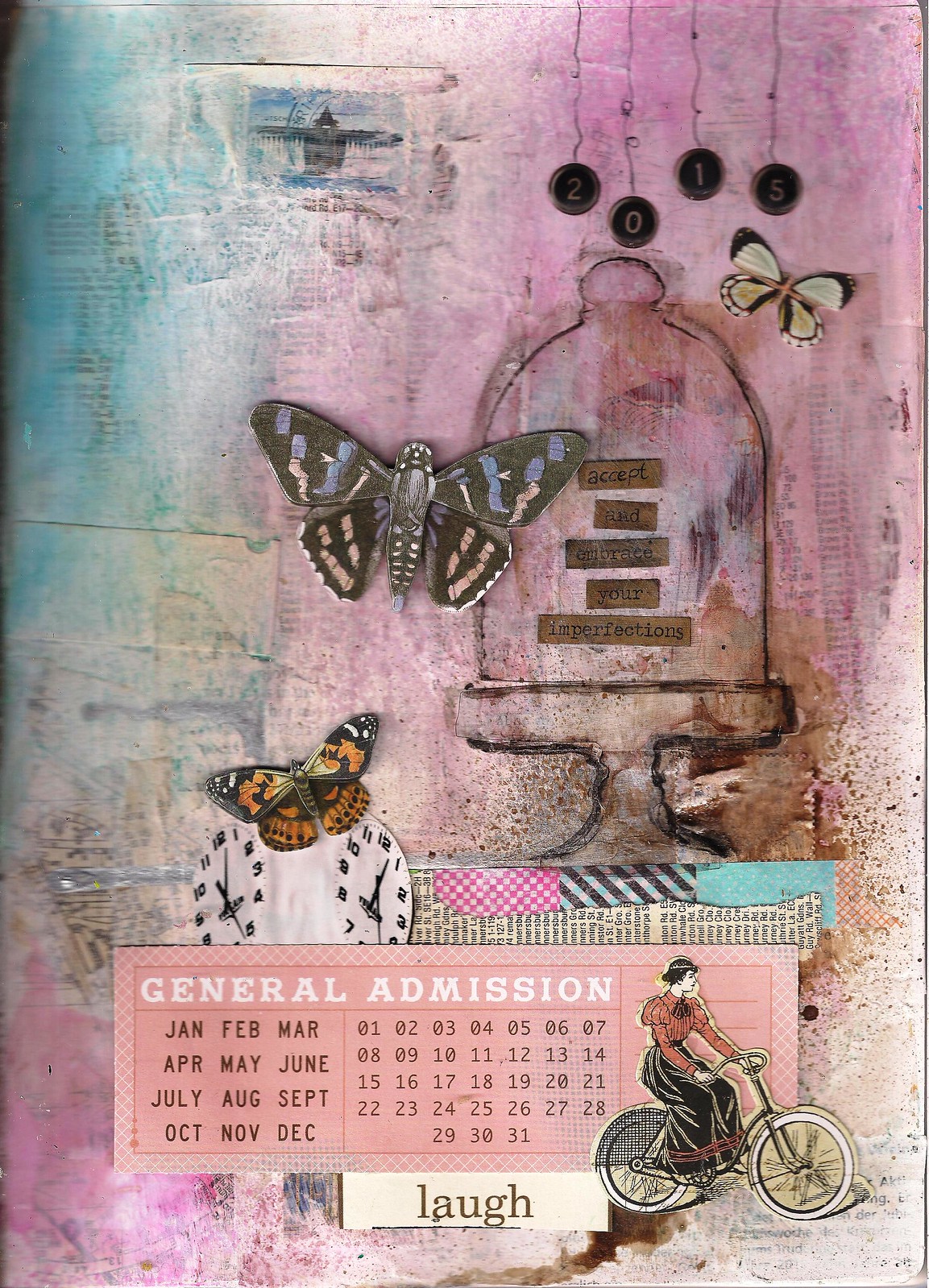This image is a highly detailed and artistic collage that appears to be a mix of various elements and media, resembling a poster or an intricate piece of artwork. The background is composed of faded newspaper pieces glued together, adorned with streaks of pastel hues in purple and blue, and splatters of brown paint concentrated more towards the bottom. 

Dangling from the upper right-hand side are four coins hanging from black strings, each bearing a digit that collectively spells out the year “2015.” Under these coins is an illustration of a glass display case, resembling a tall cake holder with a dome-shaped glass top, which has some illegible words—perhaps saying "Accept Voice Imperfections." 

Adjacent to and below this illustrated display case, there are two butterflies: one with blue and white stripes with black wings, and another in orange and black hues. Positioned below the butterflies is a white clock face with dual dials. Further down the image, an illustration of a woman in a dress riding an old-style bicycle appears, seemingly cut out from another piece and pasted into the collage.

To the bottom left of the woman riding the bicycle, there is a pink calendar-like rectangle labeled “General Admission” in white letters, displaying the months January through December and the days 1 through 31. At the very bottom of the image, a bold statement, "Laugh," is printed in brown letters on a small white background, providing a whimsical finish to this chaotic yet harmonious composition.